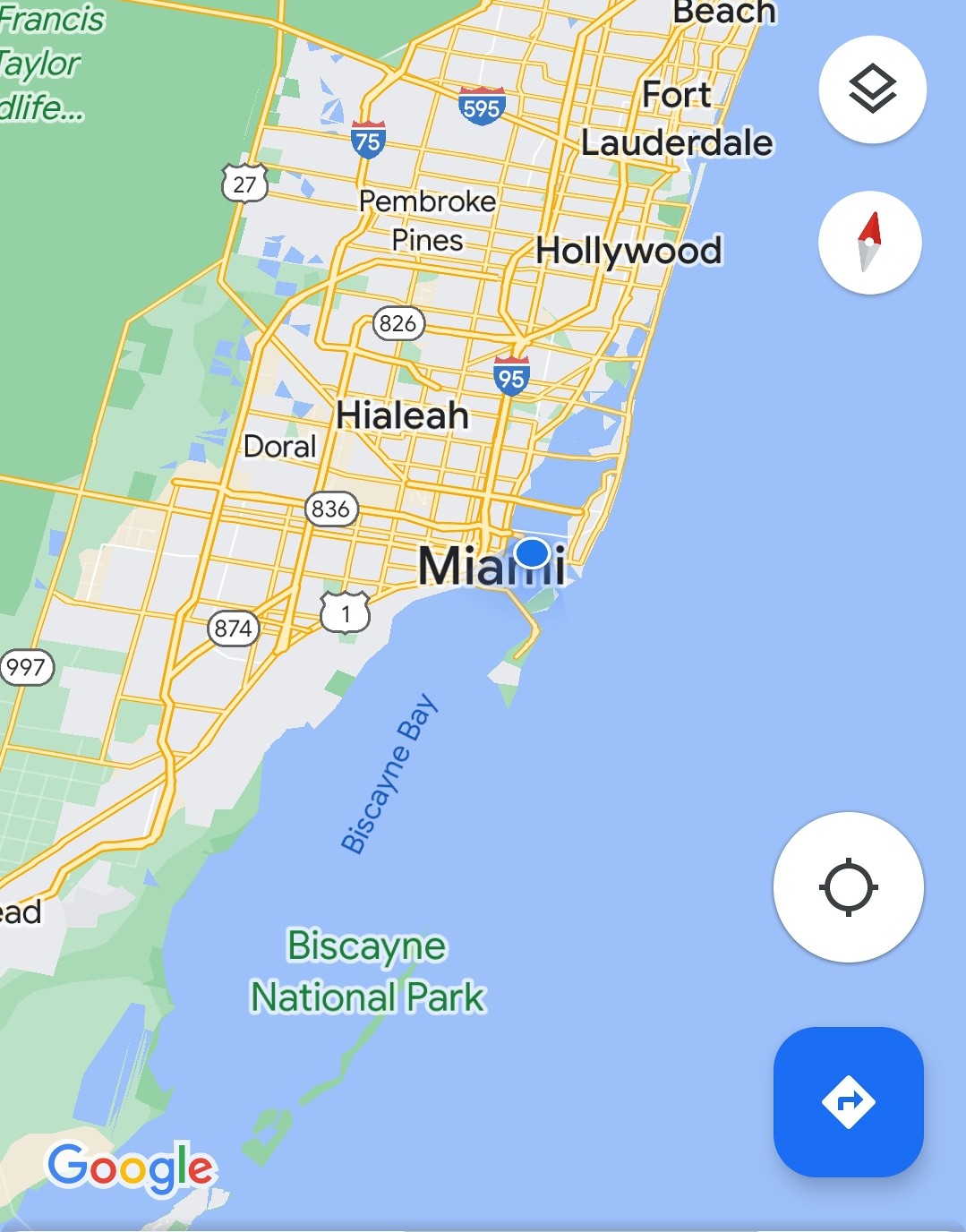This image, sourced from Google Maps, illustrates a detailed satellite view of South Florida. The water on the right portion of the image contrasts vividly with the landmass to the left. The coastline starts from the top right, approximately two inches from the edge, and follows a gently sloping trajectory to the left. Midway through, the line angles sharply leftward, before easing down again as it continues off the bottom left corner.

Along the coast is a white strip representing sandy beaches, extending approximately two inches inland, beyond which a lush green area occupies the upper left quadrant, signifying vegetated land. Interspersed within the green are yellow lines marking roads. Dense clusters of yellow lines on the white sandy strip depict city streets. Icons denoting interstates and highways are scattered throughout the map.

In particular, Fort Lauderdale is identified by its location near the northern beach area on the right side of the image. Hollywood is situated just south of Fort Lauderdale, and as the coastline makes a sharp turn, Miami appears prominently positioned. In the top right corner, a circular icon encloses a square with only the bottom visible beneath it; under this arrangement is another circle with two triangles inside, forming arrows that point in opposite directions—red upwards and white downwards.

Notably, below Miami, "Biscayne Bay" is labeled in blue, running diagonally upward to the right. Further down, "Biscayne National Park" is labeled in green. The bottom left corner of the map features the "Google" logo with alternating colors: blue, red, yellow, blue, green, and red. Finally, in the bottom right corner, a large blue square contains a smaller diamond with a blue arrow pointing to the right.

This meticulously detailed depiction represents a comprehensive view of the coastal region, capturing prominent cities, waterways, and landmarks effectively.